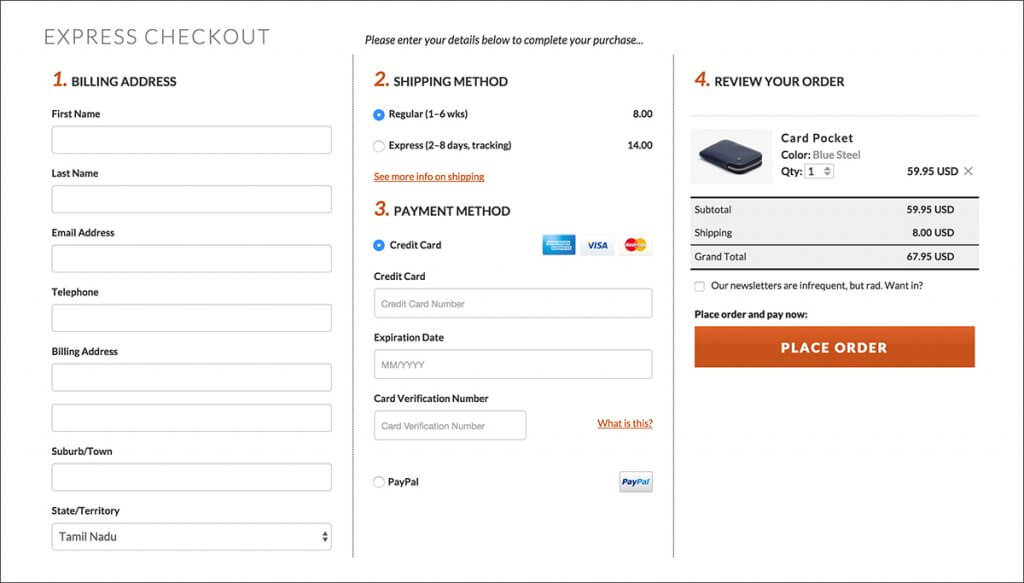The image is set against a white background, displaying a screenshot of an online checkout page. The page is contained within a light gray-bordered rectangular box. In the upper left corner, there is a vertical section titled "Express Checkout." Below this title, the page prompts the user to fill in their billing address details, which include fields for first name, last name, email address, telephone number, and physical address. The physical address fields ask for suburb or town and state/territory, with "Tamil Nadu" pre-filled in the state/territory field.

Centrally, there is a vertical prompt instructing users to "Please enter your details below to complete your purchase." Following this instruction, the page outlines the "Shipping Method" as "Regular (1 to 6 weeks)" with a cost of eight dollars indicated beneath it. The "Payment Method" section lists as number three, identified as credit card details, which include fields for credit card number, expiration date, and card verification number.

Near the bottom of the page, there is a small gray circle providing an option for PayPal, alongside the recognizable PayPal logo. On the right side of the screen, aligned vertically, is a "Review Your Order" section. This includes the item description "Card Pocket," specifying the color as "blue steel" and the quantity as one. The pricing details follow: item price at $59.95, shipping, and a grand total of $67.95 USD. Finally, in a prominent red box at the bottom, the text reads "Place Order."